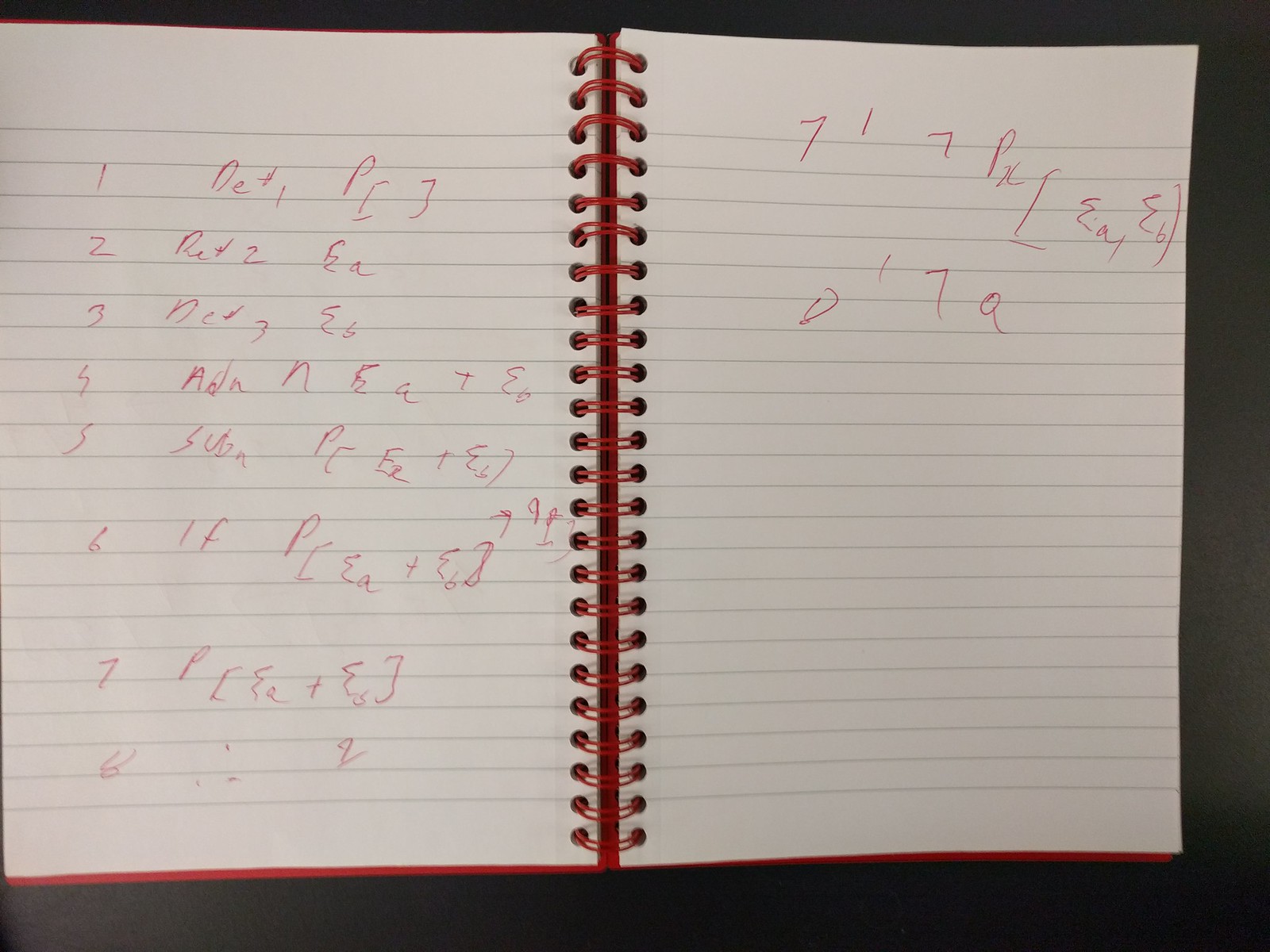The image depicts a horizontally aligned, landscape mode photograph of an open spiral-bound notebook, positioned against a solid black background that is void of any texture. The notebook, including its spiral binding, is a vivid red color. The pages are lined, clearly indicating it is meant for writing. The visible pages are covered in numerous red ink scribbles, predominantly consisting of algebraic equations. On the left-hand page, there are numbers sequentially listed from 1 to 8, each followed by various algebraic notations. The right-hand page showcases a more disordered array of numbers, concentrated towards the upper half, contributing to a chaotic yet intellectually stimulating scene.